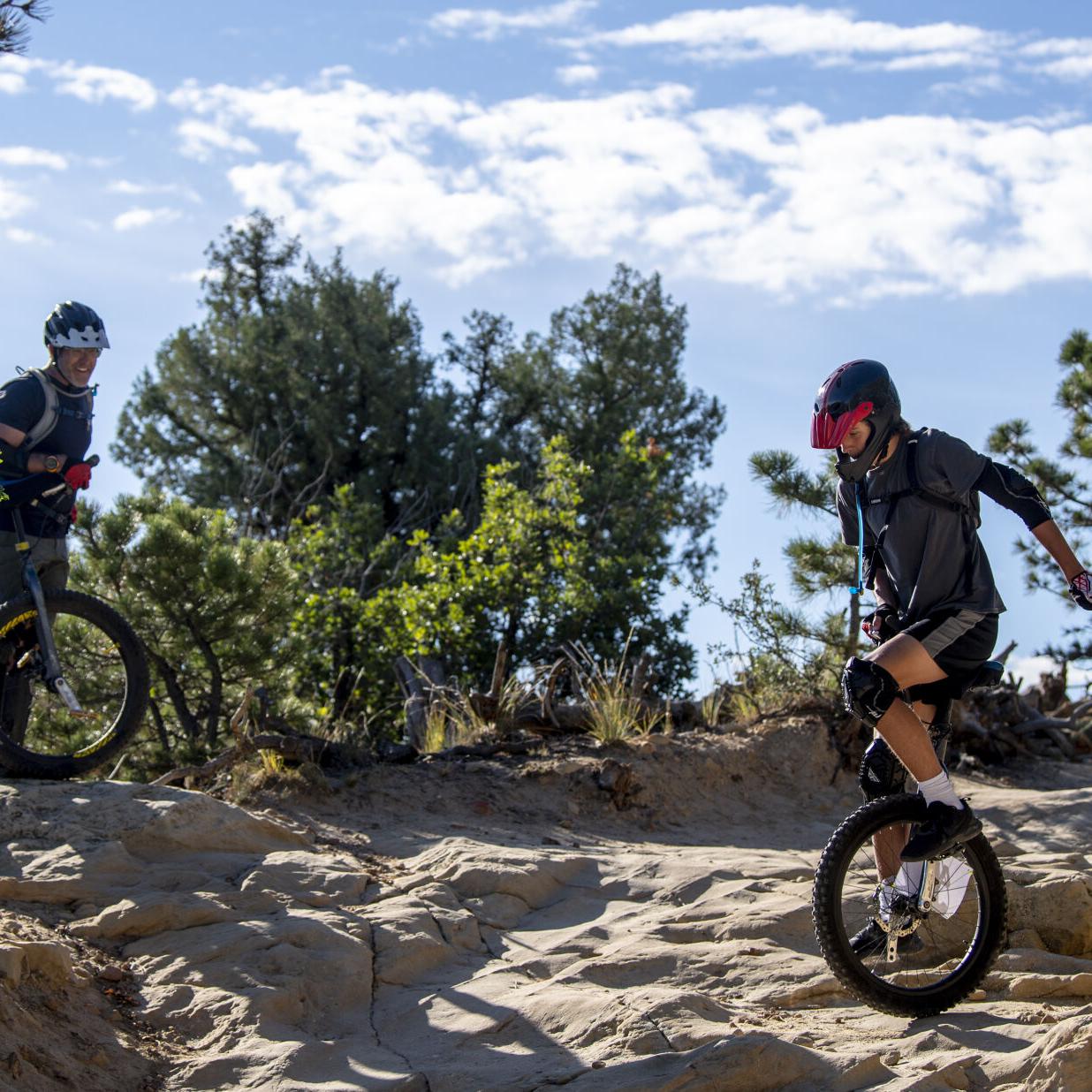In this detailed image, we observe a female cyclist on the right side riding an off-road unicycle over rugged, tan rocky terrain, likely on a mountaintop. She sports a black helmet with a red visor, black knee pads, and possibly elbow pads. Her outfit includes cycling shorts, white socks, and black shoes, and she has straps indicating something is secured to her back. Moving towards the left, she rides against a backdrop of a clear blue sky with wispy clouds. 

On the left side, a man stands beside the front tire of his mountain bike, gripping the handlebars with a gloved hand in a red glove. He wears a helmet with a light blue visor, a blue shirt, and gray pants. His mouth is open, suggesting he's smiling, and he also has something strapped to his back. Nearby, a green bush adds to the natural setting of this high-altitude adventure scene.